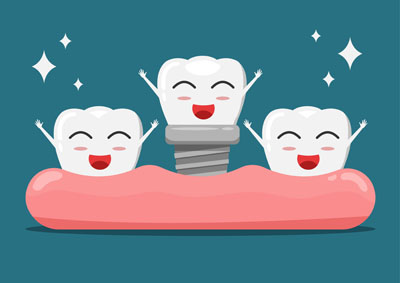The image depicts a cartoon animation of three anthropomorphized teeth, all depicted with smiling faces, blush marks, and closed eyes. Each tooth has its arms raised joyfully. The central tooth, featuring a metallic, screw-like structure below it, appears to be a dental implant and is slightly elevated compared to the other two natural teeth. These natural teeth are embedded in a pinkish-peach colored gum base. The background is a teal or dark blue shade adorned with white star-like sparkles scattered on the top left and top right. The overall scene conveys a sense of happiness and whimsy.